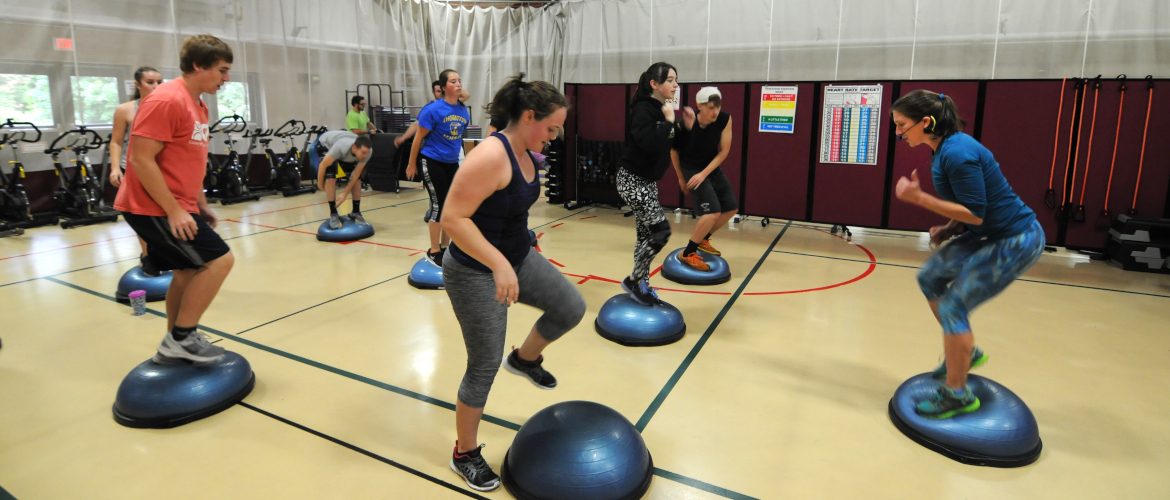In a spacious gymnasium, a dynamic exercise class is underway, featuring participants balancing on blue, dome-shaped half-balls. The scene is brightly lit by natural light streaming through several large windows, which are partially veiled by semi-sheer white curtains. The gym's wooden floor is marked with black criss-cross lines and red semi-circular lines, creating distinct zones for various activities. In the background, alongside the walls adorned with rainbow-colored posters and white and gray tiled panels, are exercise bikes and tables, further emphasizing the multifunctional nature of the space.

At the forefront, a confident and energetic female instructor stands out. Dressed in a royal blue shirt and matching patterned capri pants, she is equipped with a headset microphone, ensuring her instructions are clearly heard by the class. Her dark hair is tied back in a ponytail, and she completes her look with sneakers. Her spirited demeanor is evident as she demonstrates the workout, her thumb pointed upwards in an encouraging gesture.

Among the participants, various individuals are deeply engaged in the exercise. A woman in a black tank top and tight gray capri pants focuses intently, her left leg raised as she steadies herself on the half-ball. Nearby, a man in a peach-colored t-shirt, black shorts, and white shoes with black laces follows along, his bowl-cut brown hair slightly tousled from the activity. Another participant, attired in black and white patterned leggings and a black top, works out with equal dedication, though slightly blurred in the background.

In total, approximately ten people are partaking in the class, each with their own blue half-ball, which is flat on the bottom and rounded on top. The scene is vibrant and full of movement, capturing the essence of a modern fitness session where everyone, instructed by their enthusiastic leader, is fully immersed in their workout.